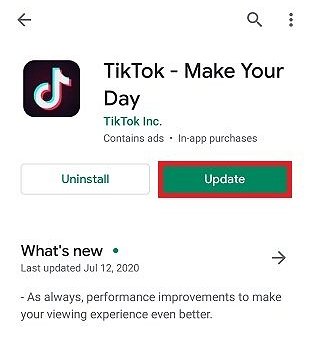This image is a detailed visual guide on how to update the TikTok app. The card features a white background, with a back arrow in the upper left-hand corner and a search icon followed by three dots in the upper right-hand corner. On the left side of the card, the recognizable TikTok icon is displayed with the text "TikTok - Make Your Day" alongside it. Directly below this, in green text, it states "TikTok Inc.".

Further down, a note indicates that the app "Contains ads and in-app purchases." Below this information, there are two buttons: a transparent button with the text "Uninstall" in green on the left, and a solid green button with the text "Update" on the right. The "Update" button is conspicuously outlined in red to draw attention, emphasizing the focal point of the guide.

Additionally, the card includes a section titled "What's New" with a small green dot, informing users that the app was last updated on July 12th, 2020. Underneath this are the details of the update, mentioning "As always, performance improvements to make your viewing experience even better." A right arrow placed below this information suggests further details or navigation.

The overall purpose of this card is to instruct users on how to update their TikTok app. The creator has marked the update button in red to effectively guide TikTok users, possibly followers of their own TikTok account, on getting the latest and best viewing experience by keeping the app updated.